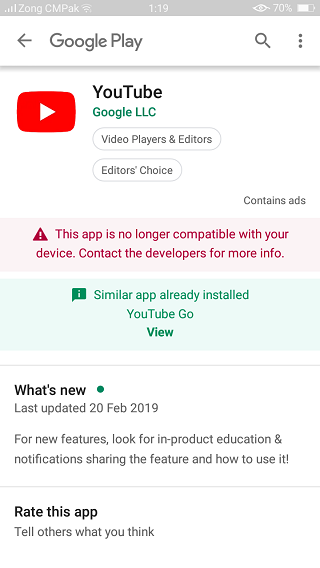A detailed screenshot of a mobile app interface is displayed, shaped vertically in a rectangular form, typical of a mobile device screen. The top portion of the screenshot is a gray status bar. On the left side of the status bar, it reads "ZONG CMPAC," accompanied by four or five signal bars and a Wi-Fi icon, signifying connectivity status. Centrally located in this bar, the time is displayed as "1:19." On the right side, there is a 70% battery icon and an eye-shaped icon.

Directly below the status bar, there is a search box labeled "Google Play," characterized by a white background with a magnifying glass icon on the left, indicating its search functionality.

The main content starts underneath the search box, with "YouTube" and "Google LLC" centrally displayed, set against a white background. 

To the left of "YouTube" and "Google LLC," there is the familiar YouTube logo – a red rectangular box with a white play button (a triangle) inside. It labels the app as a "video players and editors" category and marks it with an "Editor's Choice" badge.

A prominent pink text box just below states, "This app is no longer compatible with your device. Contact the developers for more information," with the text in a slightly deeper red shade. 

Beneath that, a green text box notes, "Similar app already installed: YouTube Go," with a "View" button highlighted in green text.

Following these announcements, there are sections titled "What's New" and "Rate This App," each providing brief information. The "What's New" section mentions the last update date as "20 February 2019."